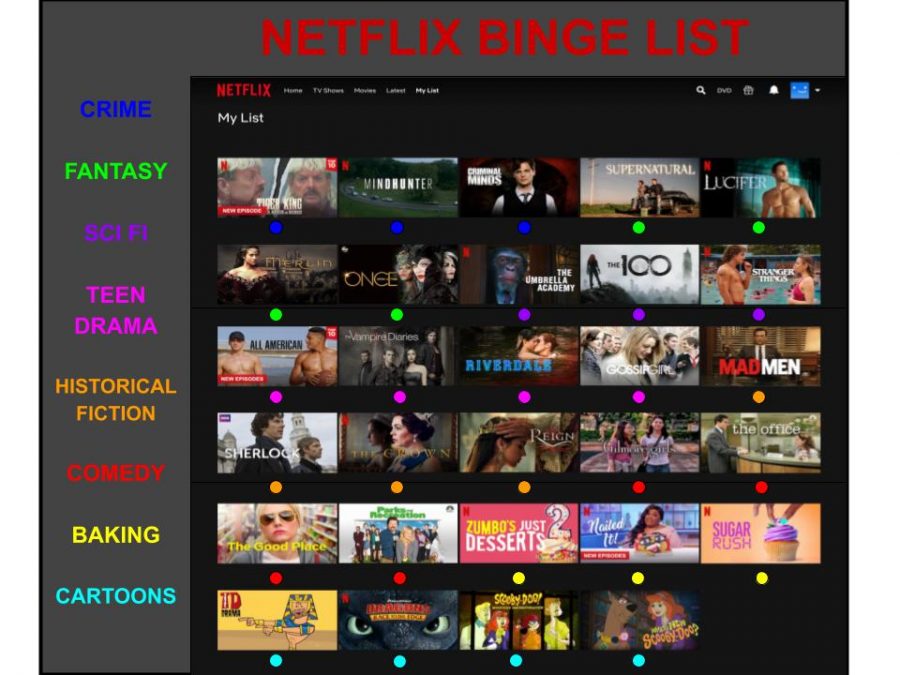A detailed screenshot reveals a customized list of Netflix movies and shows, organized in a manner reminiscent of a tier list but designed to reflect personal viewing priorities and genre classifications. The compilation includes titles such as "The 100," "Once," "Riverdale," "Zombo's Just Desserts 2," "Total Drama Island," "Mad Men," and "Stranger Things." Each item is categorized under distinct genres listed on the left side of the screenshot, which are: crime, fantasy, sci-fi, teen drama, historical fiction, comedy, baking, and cartoons. For example, the 'cartoons' genre, marked by bright blue text and blue circles under each title, includes "Total Drama Island," "How to Train Your Dragon," and "Scooby-Doo." Similarly, the 'historical fiction' genre, identified by orange text, features titles such as "Mad Men." This color-coding system clearly indicates the user's personalized sorting methodology, providing both an aesthetic and functional means of organizing their viewing preferences.